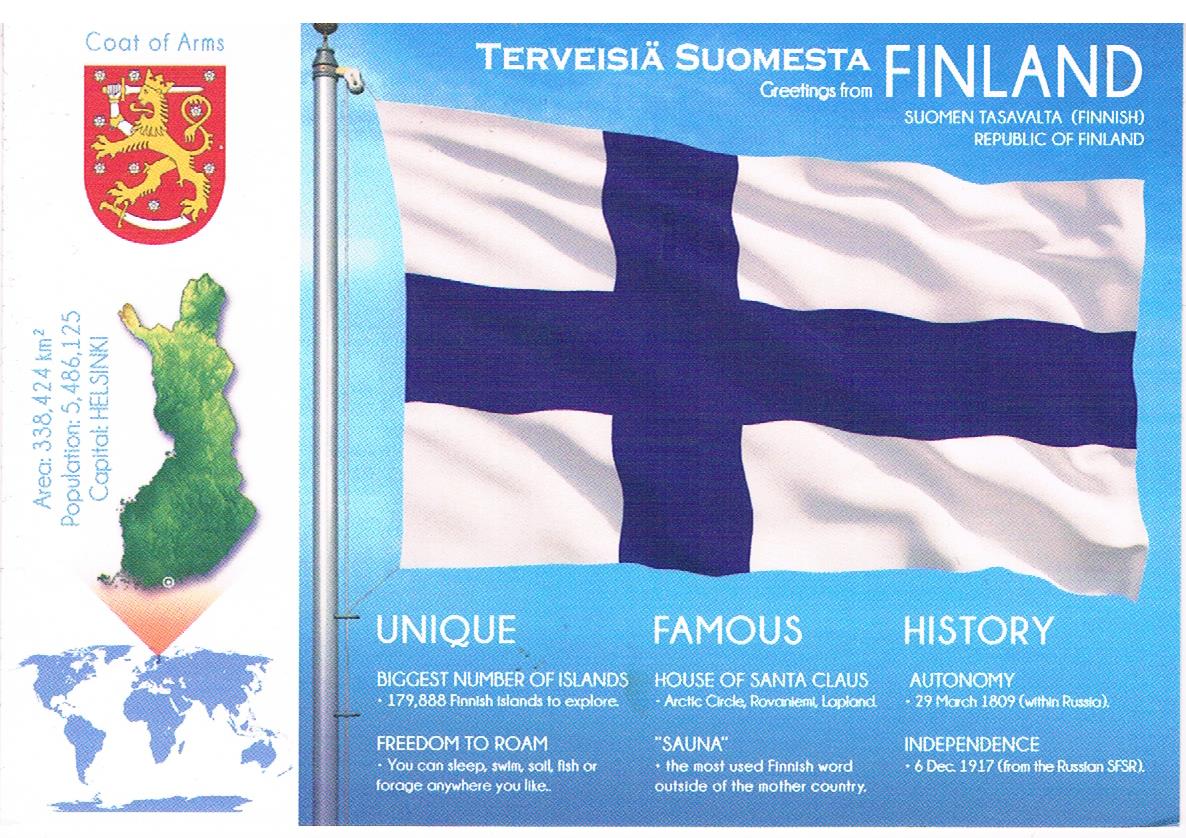The image provides intricate details about Finland. At the center is the Finnish flag, featuring a white background with a blue cross. On the left side of the flag, there is Finland’s coat of arms, characterized by a red shield with a crowned yellow lion holding a sword. Above the flag, text reads "Greetings from Finland" in Finnish, with "Republic of Finland" also noted. The right side of the image highlights key aspects of Finland, such as its status as having "the biggest number of islands" (179,888 in total) and the "freedom to roam," allowing activities such as sleeping, swimming, sailing, fishing, or foraging freely across the country. The section also mentions notable features like the house of Santa Claus in Lapland, the Arctic Circle, and the nation’s famous affinity for saunas. 

Further details include historical points such as Finland's autonomy on March 29, 1809, and its eventual independence from Russia on December 6, 1917. Additionally, there is a small map of Finland, highlighting its area of 338,424 square kilometers, a population of 5,486,125, and its capital, Helsinki. At the bottom, a world map is shown for context. The entire depiction provides a comprehensive overview of Finland’s geography, history, and cultural highlights.